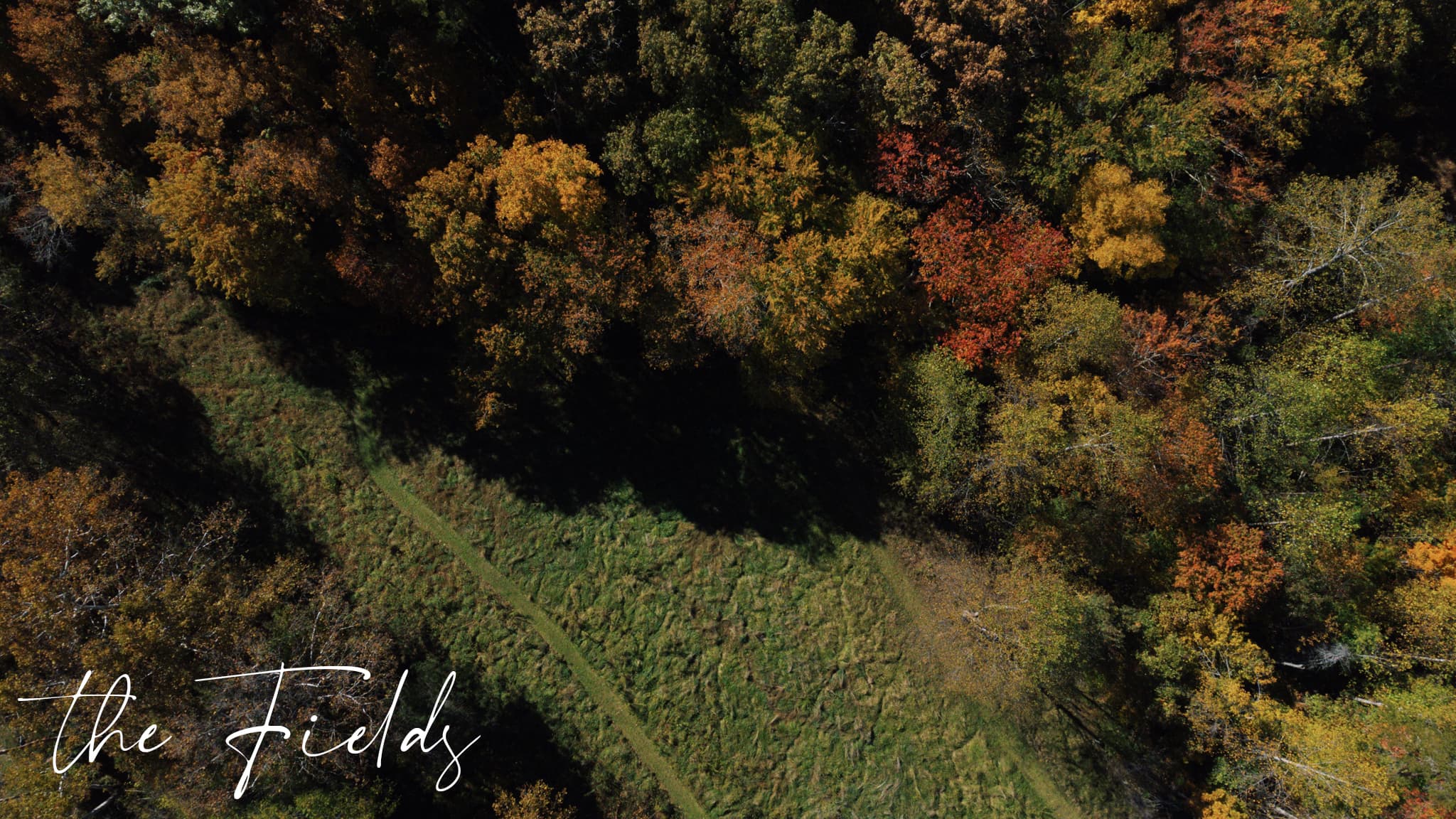An aerial painting-style image captures an autumnal forest with vibrant fall foliage, predominantly featuring red, orange, yellow, and green trees. The landscape layout allows for a comprehensive view of the scene, resembling a view from an airplane. A striking wedge of green trees runs diagonally from the top left to the middle bottom of the image. The lower left-hand corner of the painting displays the phrase "the fields" in white cursive. This area appears grassy, potentially a walking path or cleared trail, enhancing the natural beauty of the setting. The right side and upper half are dominated by clusters of colorful trees, while the lower right showcases a darker patch where some trees have shed their leaves, adding to the rich tapestry of autumn colors. The overall composition exudes a serene yet dynamic autumn landscape with washed-out colors, emphasizing the seasonal transition.